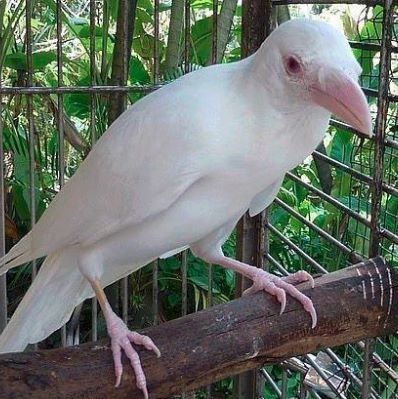The close-up image depicts a large, white bird, likely a parrot, inside a wire mesh cage. The bird is perched on a brown branch that runs through the middle of the cage. Its feathers are entirely white, and it has a pinkish beak and pink claws, with the central claw being longer than the two on the sides. You can see the bird’s right eye, which appears to be predominantly brown but may have a reddish or pinkish tint. The bird is staring directly at the camera. Surrounding the cage are various trees with large, sweeping, and spiky green leaves, creating a lush backdrop.